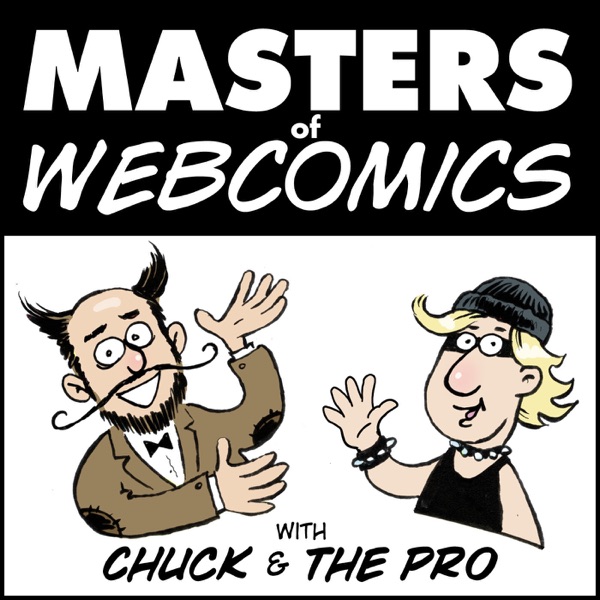This nearly square poster advertises internet comics, titled "Masters of Webcomics." The top third of the poster features a solid black background with large white letters: "MASTERS" in thick, bold font, followed by "OF" in smaller font directly beneath it, and concluding with "WEBCOMICS" in a slightly smaller, different font. The lower two-thirds of the poster displays two cartoon characters. The character on the left is a man dressed in a brown suit coat with black patches on the sleeves, a white shirt, and a black bow tie. He has a prominent handlebar mustache, a beard, and hair on the sides of his head. The character on the right wears a black beanie hat, a black mask over his eyes, a black tank top, and accessories that include a studded bracelet and necklace. This character also has long blonde hair. The bottom of the poster features additional text, with "WITH" in smaller letters followed by "CHUCK AND THE PRO" in larger, bold letters.